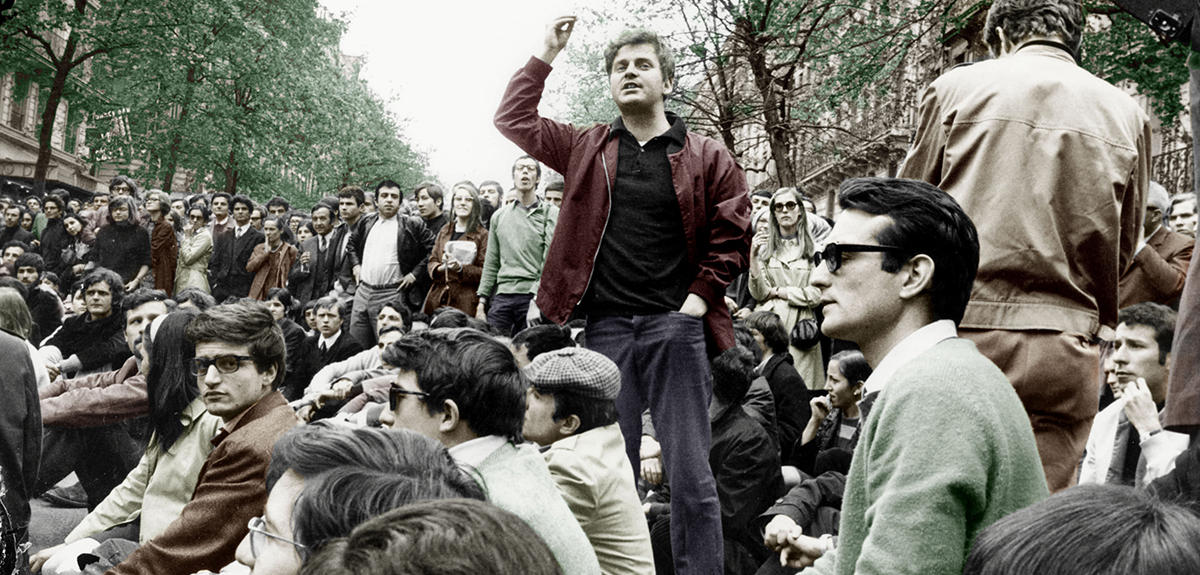This photo appears to depict a large outdoor gathering from the 1960s or 1970s, possibly in a European city like France, Germany, or England. The assembly comprises predominantly young people, mostly men, seated and standing along what seems to be a tree-lined city street, with lush green foliage framing the scene. The colors in the image are slightly washed out, adding an old-fashioned feel. Dominating the center of the photo is a man in a red jacket, black shirt, and gray pants, standing with his left arm raised, while his other hand rests in his pocket. He appears to be speaking to the crowd, which is focused intently on him. A man beside him, possibly older, is turned away, looking down and wearing a tan coat and pants. The gathering seems significant, though the exact nature of the event remains unclear from the image alone. The overall impression is that of a peaceful public assembly or protest.